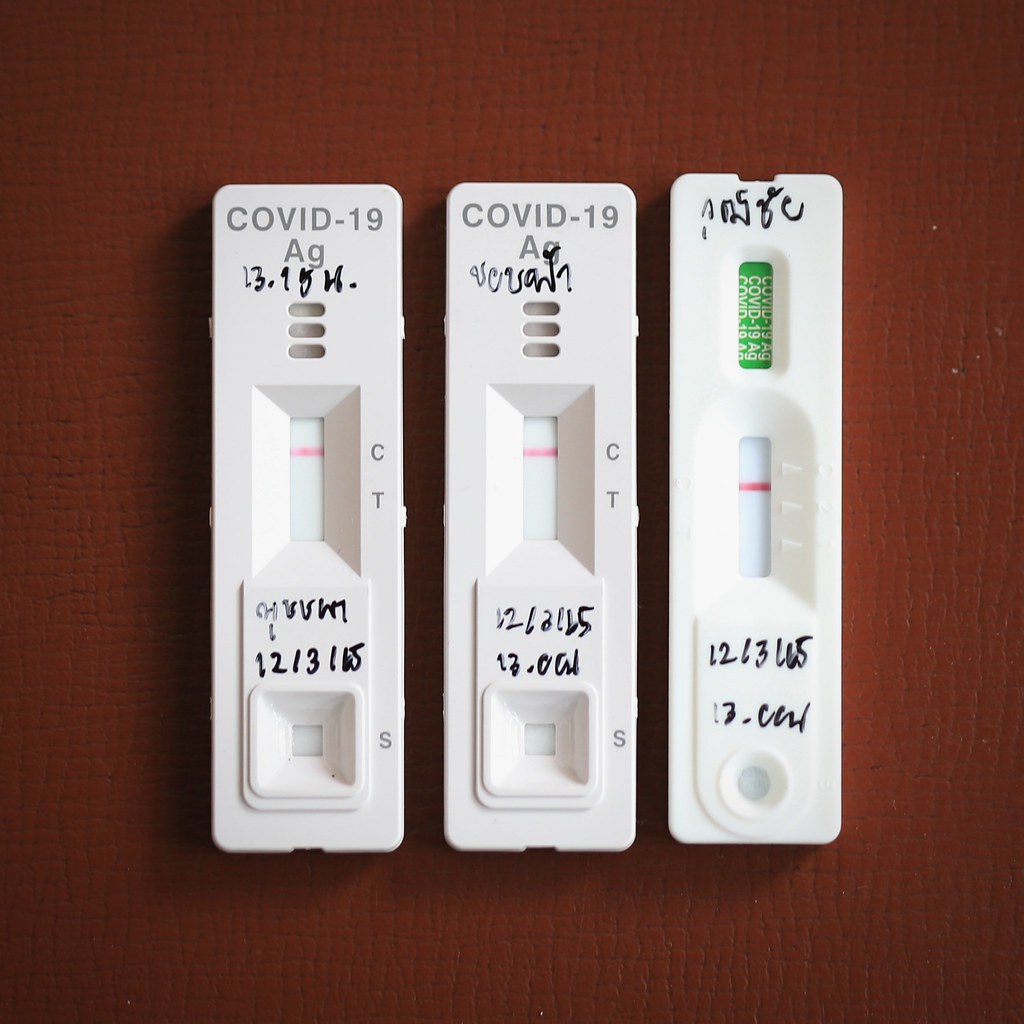The image is a square photograph featuring three COVID-19 test kits positioned vertically against a purple fabric background. The two test kits on the left and center are identical in design. They are white and contain several distinctive features. At the top, each kit has three small, capsule-shaped openings. Below these is a trapezoidal indentation with a horizontal line marking at the bottom. Further down, there is a small square opening within a larger, slightly raised square area. Handwritten in Sharpie, above the main testing area labeled “COVID-19 AG,” are various numbers or letters. Underneath the central trench-like testing region, the values “C” (Control) and “T” (Test) are marked, with the control line showing a red mark while the test line shows none, indicating negative results.

The test kit on the right differs in design. It has a rectangular shape and two openings. The top one bears green coloring with white lettering that reads "COVID-19 AG." Below this, a red control line is visible in a rectangular window, and the bottom section features a circular area designated for placing the test sample. The contrasting designs and specific markings clearly highlight the differences between the two kinds of test kits displayed in the image.